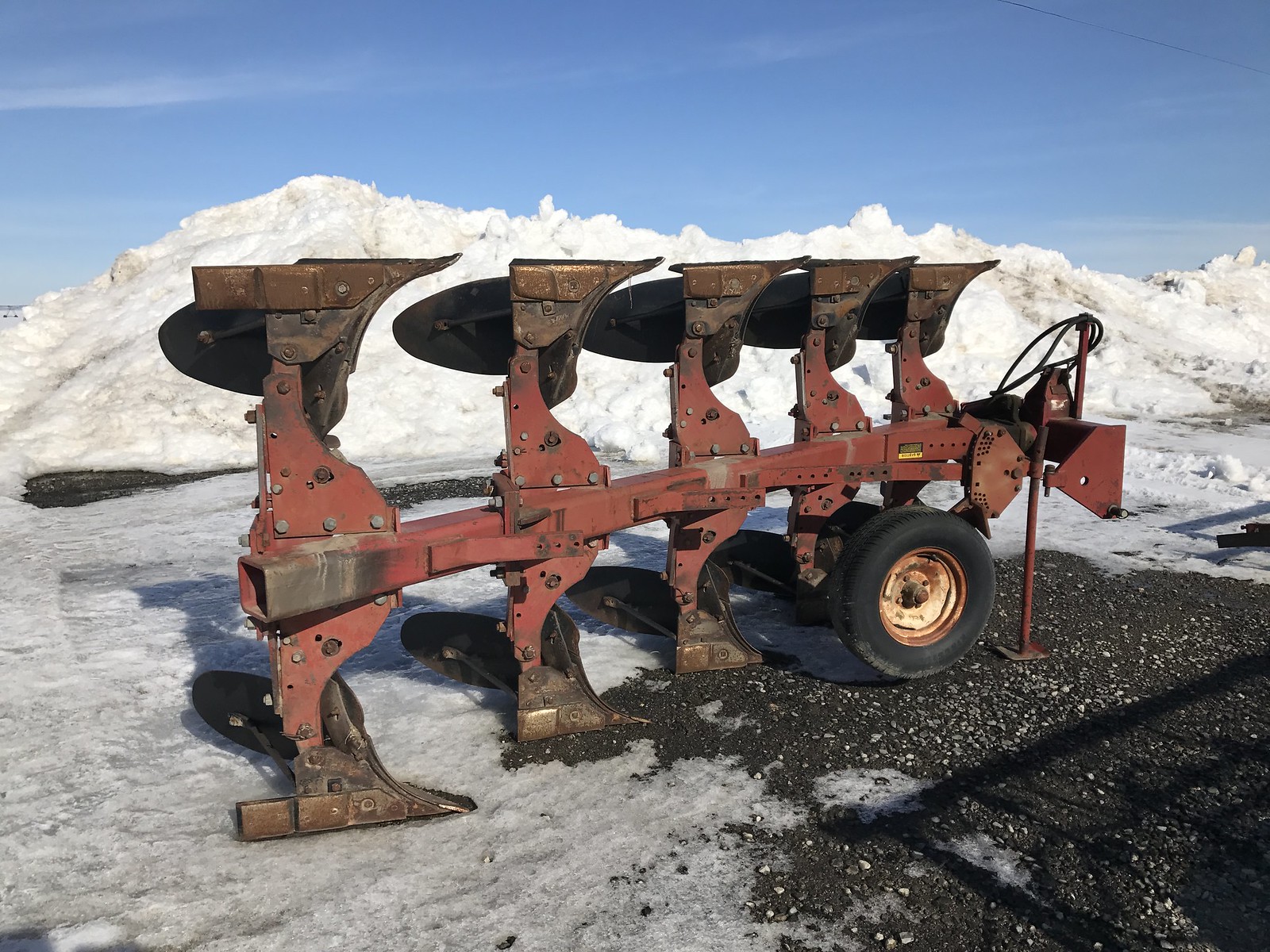A color photograph captures a maroon steel trailer attachment with rust-colored ends, seemingly designed for a larger truck. The trailer, which appears to be flipped on its side—a position that might be intentional—features one visible black tire on the ground and several steel structures, including a supporting pole with rope possibly used for pulling. The scene is set outdoors in the daylight, with a clear sky dotted with a few clouds. The trailer rests on a black gravel and snow-covered pavement, partly cleared but with some residual snow and salt around it. A large snow pile serves as the backdrop, emphasizing the wintry conditions of the setting.